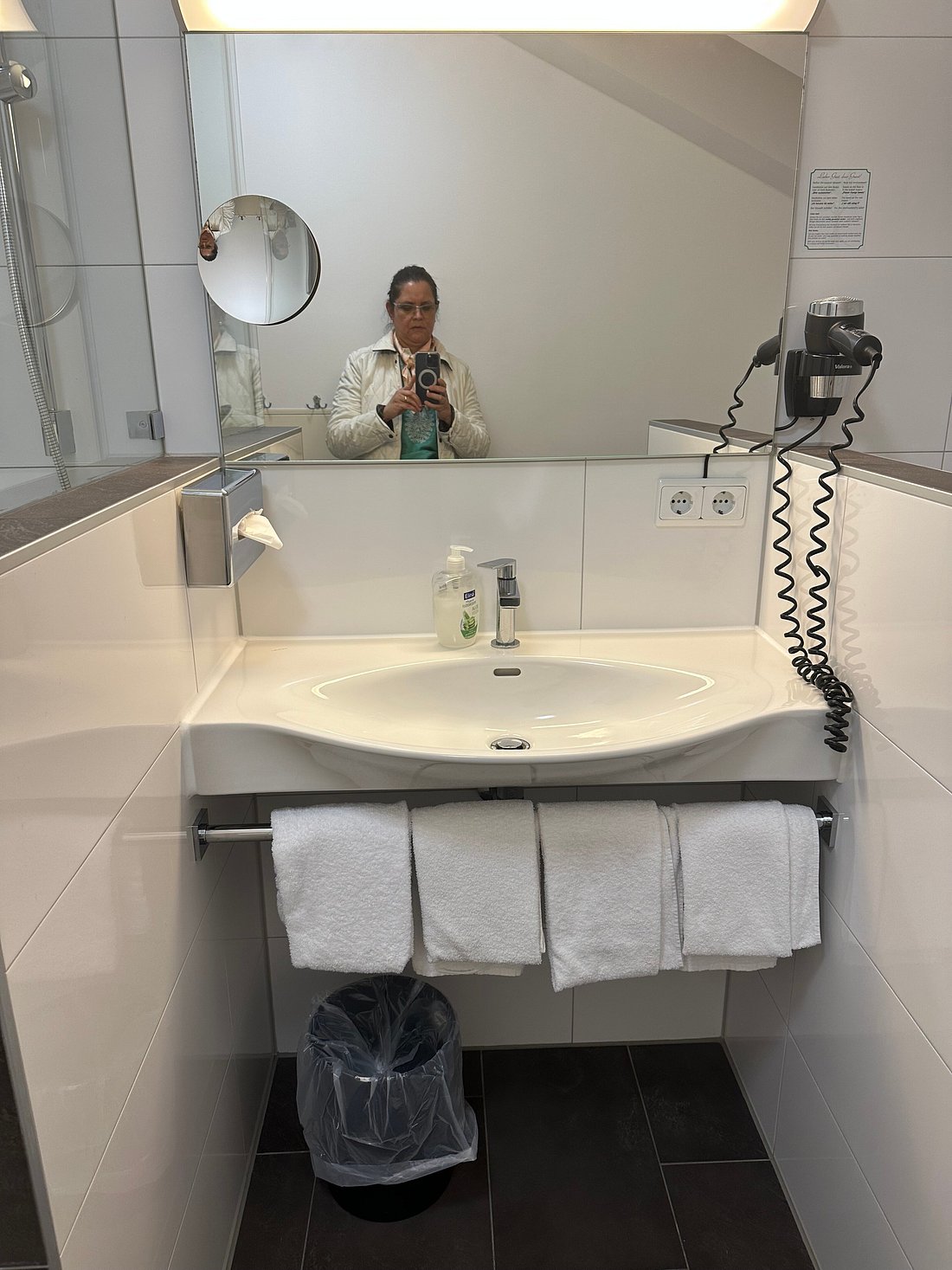This photograph captures a detailed scene within a well-appointed bathroom, likely in a hotel. Central to the image is a porcelain sink with a faucet resembling an old-fashioned well pump, complemented by a bottle of hand soap. Above the sink, a large mirror with an oval magnifying section is illuminated by a fluorescent light fixture. The bathroom features white tiled walls and contrasting black tile flooring. A metal Kleenex holder is mounted on the left wall, while a hair dryer hangs from a hook on the right.

Below the sink, a metal rod supports four folded towels, and beneath that, a black plastic-lined trash can is placed. Adjacent to the sink there is a glass-walled shower visible on the left side of the frame. The focal point of the image is a woman, likely in her forties, dressed in a blue shirt and a white jacket, with her hair pulled back and wearing glasses. She stands in front of the sink, holding up an iPhone to take a selfie.